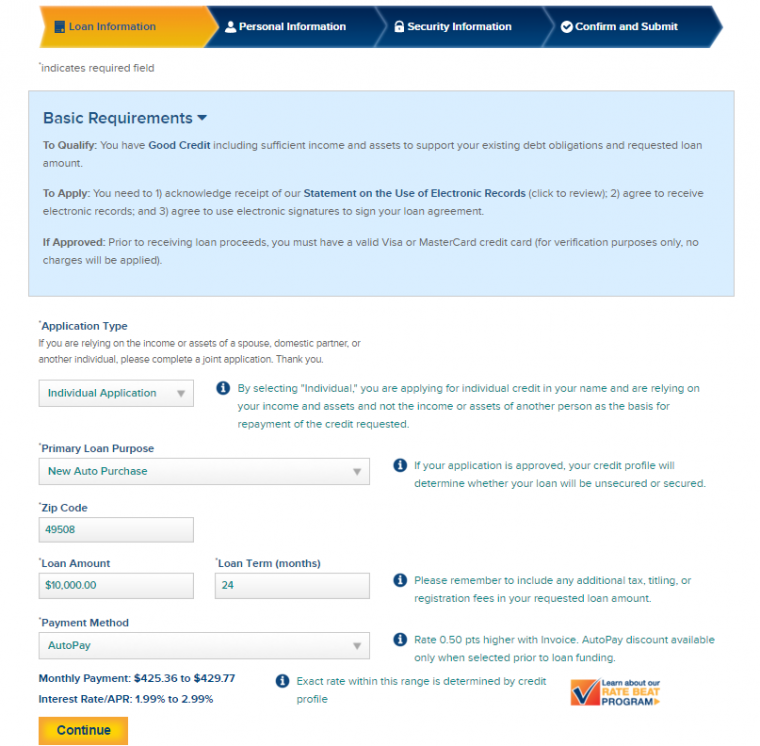The image depicts a webpage showing a loan application interface. The webpage has multiple tabs positioned at the top, with "Loan Information" currently selected and highlighted in orange. The other tabs, colored in dark blue, are labeled "Personal Information," "Security Information," and "Confirm and Submit." 

Beneath the tabs, there is a section that contains a note about required fields, indicated by an asterisk. Below this note, a light blue box titled "Basic Requirements" is visible, accompanied by an arrow pointing to a list of basic requirements for the loan. Following this, there is a form section where users can input their information, including details on monthly payments and interest rates. At the bottom of this section is an orange button labeled "Continue."